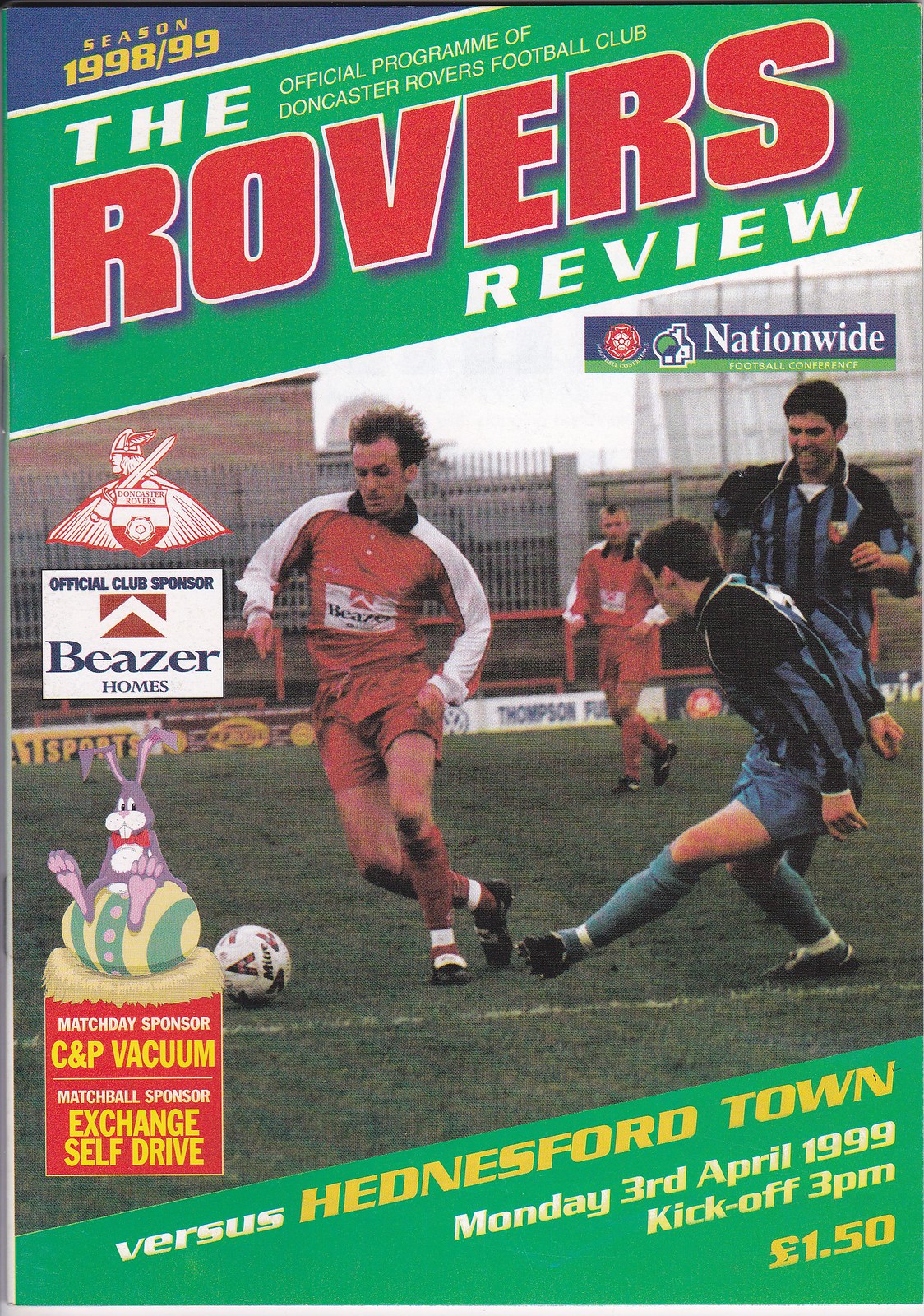The cover of the magazine, titled "The Rovers Review Season 1998-99," serves as the official program of the Doncaster Rovers Football Club. Prominently displayed at the top are its major sponsors: Nationwide Football Conference and Beezer Homes. Additionally, the program is supported by match day sponsor C&P Vacuum and match ball sponsor Exchange Self-Drive. A distinctive Viking emblem holding a sword is also present. In a festive touch, an Easter-themed image features a pink rabbit sitting on a colored egg. At the center, an action-packed photograph captures four players in the midst of a soccer match—two in red and white jerseys, and two in black and silvery blue—chasing a soccer ball. The bottom right corner of the cover details the upcoming match: Doncaster Rovers versus Hednesford Town, scheduled for Monday, April 3, 1999, kicking off at 3 p.m., with an entry price of 150 pounds.